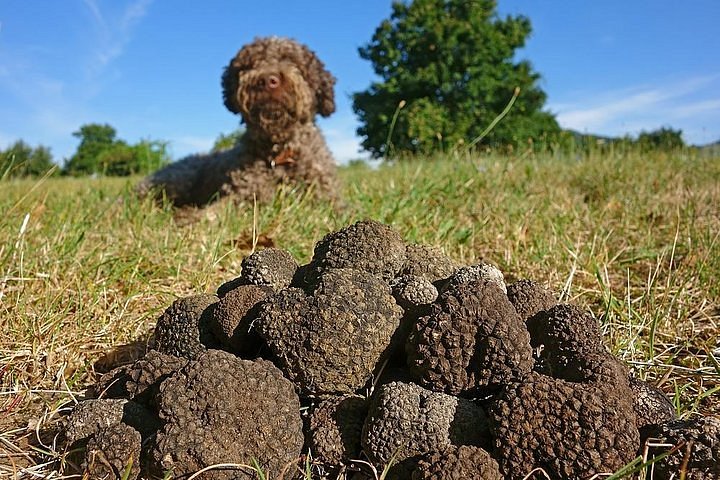This landscape-oriented color photograph captures a detailed outdoor scene on a bright, cloudless day. In the foreground, there is a collection of black and brown rocks of various sizes and shapes. Among these rocks are some substantial chunks interspersed with smaller stones, creating an intricate, stacked arrangement at the bottom center of the view. Rising above these rocks, a lush grassy field extends towards the horizon. 

At the center of the image, a fluffy toy dog, likely a Bernedoodle, lies on its stomach among the grass. This brown dog sports light curly hair largely covering its face, obscuring its eyes. The dog's head is lifted, looking directly towards the viewer. In the background, beyond the dog and grassy field, several green trees are visible, with one particularly prominent tree almost centered in the image. 

The overall theme is one of natural realism, capturing the serene and vivid elements of the landscape with an emphasis on the contrasting textures and colors of rocks, grass, and the dog's fur.